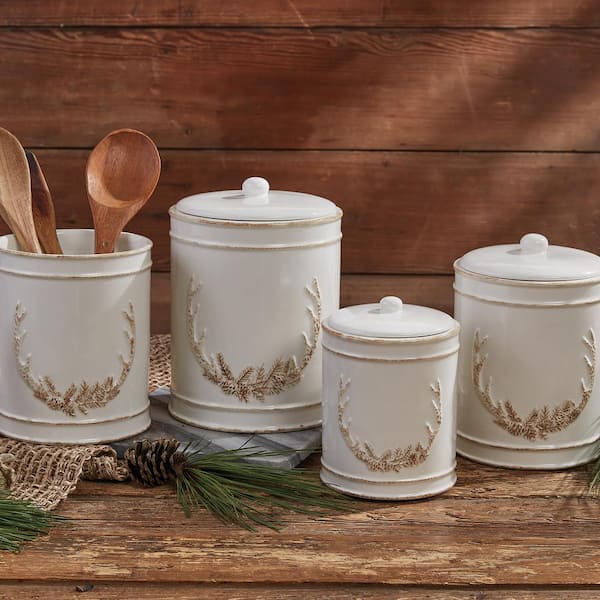The photograph showcases four cylindrical kitchen canisters, predominantly white with a tan and brown antler design made of stylized pine branches on the front of each. These canisters, likely made of metal, are arranged on a heavily weathered wooden table against a similarly weathered, cedar-colored wooden wall, evoking a rustic, cabin-like atmosphere. The surface of the table is adorned with pine cones, pine needles, and a strip of canvas cloth, which add to the natural and cozy aesthetic. The canister on the far left has its lid removed, revealing three large wooden kitchen utensils, including ladles and spoons, while the other three canisters remain covered with traditional lids featuring central knobs. Patches of sunlight or artificial light gently illuminate the scene, highlighting the textures and enhancing the warm, homely feel of the composition.